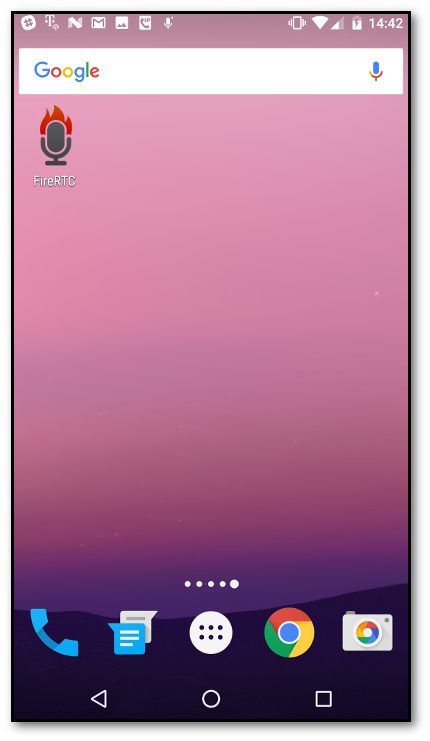The image is a meticulously detailed graphical representation of a smartphone interface. At the top of the screen, there are various status icons including cell signal strength, Wi-Fi signal, battery level, and the time displayed as 14:42. Just below these icons lies a uniquely shaped search bar. It is white with the word "Google" written in the traditional colorful font, and features a microphone icon on the right side, indicating voice search functionality.

The phone's background starts with a soft mauve color at the top that gradually transitions to a darker mauve and finally to a deeper purple, depicting a serene gradient. At the very bottom, the gradient meets a slight hill-shaped silhouette and stars scattered in the backdrop, ranging from red to purple hues, enhancing the visual allure.

Underneath the search bar, the phrase "Fire RTC" is prominently displayed with both "F" and "RTC" capitalized. Adjacent to this text is a cartoon-style microphone icon with flames at the top, reinforcing the brand's fiery theme.

On the screen's interface, at the bottom, four distinct icons are neatly arranged. These include a telephone icon, a messaging icon, a circular icon with six dots (representing apps), the Google Chrome web browser icon, and a camera icon. Notably, the camera icon intriguingly incorporates the Google Chrome logo within it.

Additionally, the primary phone icon at the very top is outlined in a square shape with soft, rounded edges. The interior of this square contains various elements including a hashtag symbol, and letters "T", "N", and "M" within distinct white squares. A further square depiction includes miniature icons such as a stylized mountain image, a traditional telephone symbol marked "IP", and another microphone icon. This describes the intricate and multifaceted design of the smartphone’s home screen.